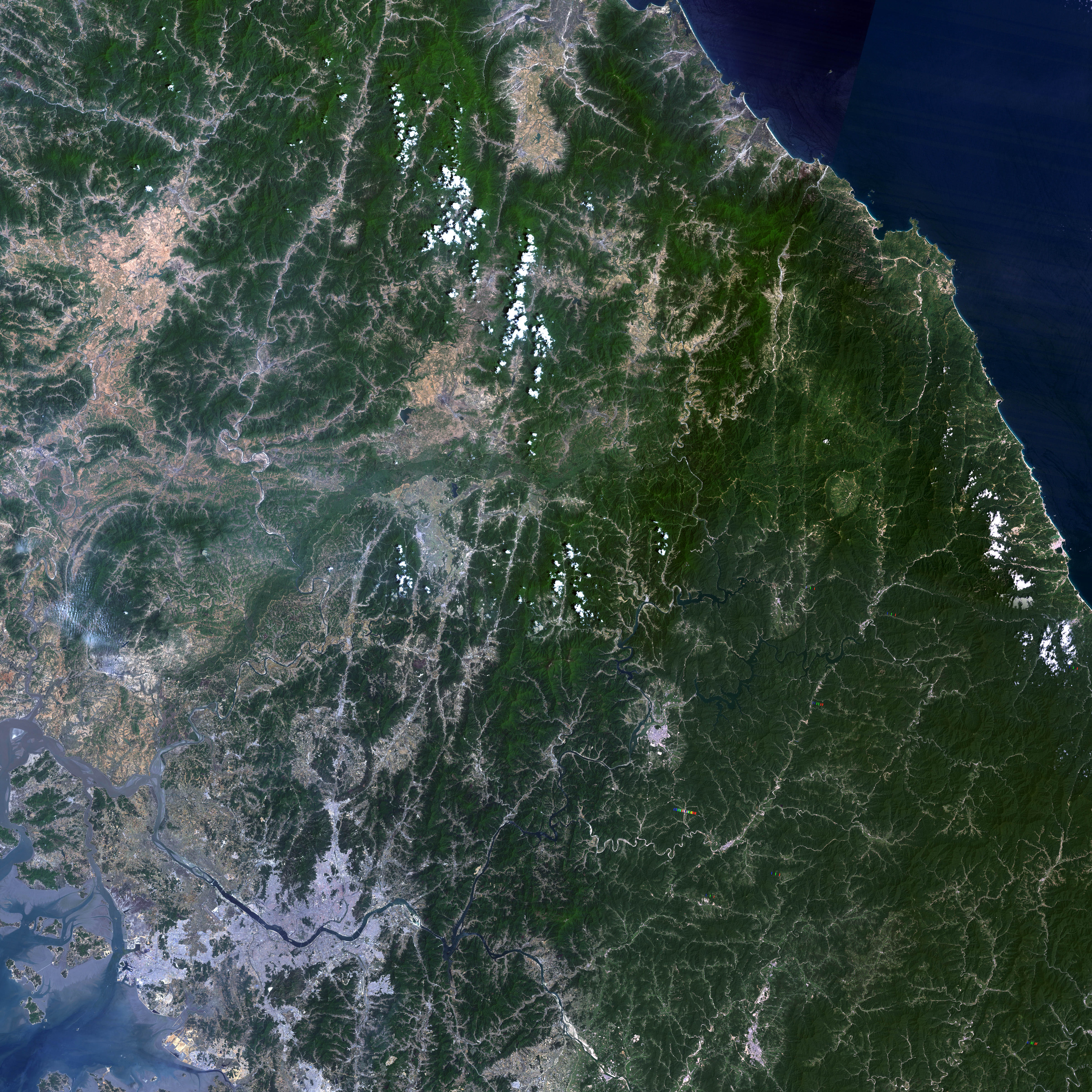The image appears to be an aerial photograph or satellite image of a coastal region, possibly taken from outer space. Dominated by lush greenery, it showcases a diverse terrain. The top right corner features a dark blue expanse that appears to be the ocean, with a coastline marked by dark green edges. The landmass reveals intricate details, including cracks and white patches, possibly representing rivers or snow. Towards the bottom left corner, the landscape shifts to gray with swirls of blue, indicating rocky or stone-filled areas and water bodies. Brown regions scattered throughout may represent mountains or sandy areas. The overall terrain seems to be a mountainous forest area, rich in natural features and bordered by water, making it likely a coastal forested mountain range captured from a high altitude.